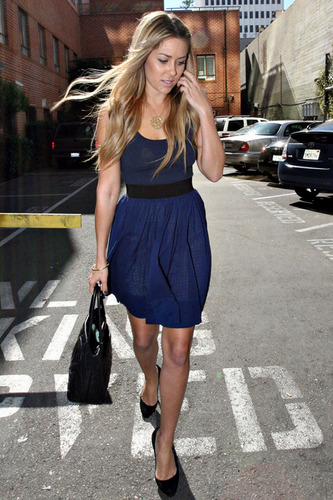In the small vertical rectangular image, a woman is captured mid-stride as she crosses a parking lot road. She is dressed in a sleeveless, navy blue sundress that features a black belt cinching her waist. Complementing her outfit, she is wearing black high heels and a gold chain necklace ending in a circular pendant, along with a gold bracelet on her right wrist. She carries a black handbag in her right arm while her left arm is bent toward her face, lightly touching her long, slightly wavy blonde hair, which flows over her shoulders and is rustled by the wind. She gazes downward towards the bottom right of the image as she walks over white pavement lettering, likely indicating parking information.

In the background, the scene unfolds with multiple cars parked along the grey asphalt surface. To her left, the taillights of a pickup truck can be seen, while behind her, a mix of architectural elements form a diverse urban landscape. On the left side is a two-story brown stone building with rectangular windows, and to the right is a red brick structure with a white awning. Further in the distance, a white stone building is visible, along with glimpses of the sky and trees, adding depth to the image.